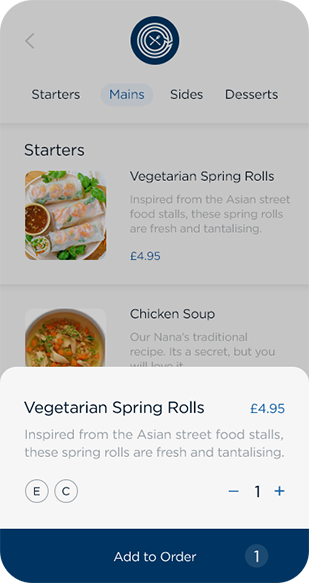The image depicts an online food ordering interface. At the center, a blue circle contains white icons of a fork and knife, indicating a food service theme. Above, there is a back arrow. Below this iconography, the categories "Starters," "Mains," "Side Dishes," and "Desserts" are listed, with "Mains" being highlighted.

The "Mains" section features two items. The first is "Vegetarian Spring Rolls," described as taking inspiration from Asian street fair stalls, promising freshness and tantalizing flavors, priced at $4.95. The second item is "Chicken Soup," labeled as "Nana's Traditional Recipe," boasting a secret, heartwarming flavor, illustrated with a picture of the soup.

Under these descriptions, there is a control bar for ordering. It includes the dish name “Vegetable Spring Rolls” once again, accompanied by the same enticing description about their freshness and Asian street food inspiration. To the right, within circles, are the letters "E" and "C" perhaps indicating dietary information. A numeric adjustment feature allows users to specify quantity with a plus or minus button and the current selection set to one. 

At the bottom of the interface is a prominent blue bar labeled "Add to Order" in white text, signifying the option to add the selected item (currently one spring roll) to the order.

Overall, the image portrays a digital menu from which users can conveniently select and customize their meal choices.